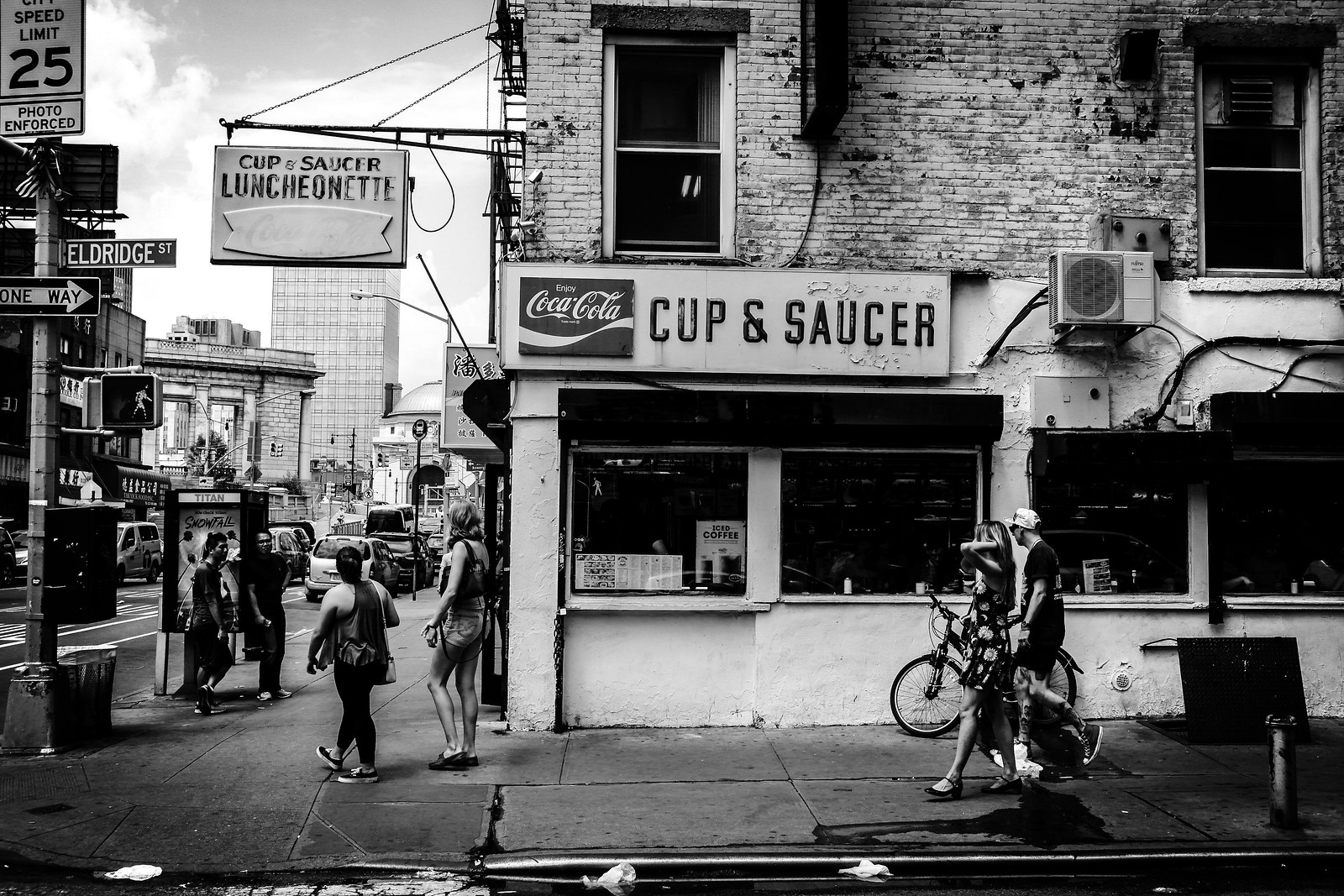This black-and-white photograph captures a bustling street corner, likely located in the Lower Manhattan area, evidenced by what appears to be the entrance to the Manhattan Bridge in the background. The scene, possibly from the 1960s or 70s or edited to appear that way, showcases a gritty urban landscape under a cloudy midday sky. Prominent in the foreground is the Cup and Saucer luncheonette, an old brick and cement building with a faded, whitewashed facade. Above the entrance, an outdated sign featuring a Coca-Cola logo invites patrons to "Enjoy Coca-Cola."

The intersection is teeming with life; seven pedestrians navigate the wet, litter-strewn sidewalks amidst traffic. One man walks his bicycle, while a woman in a short, loose-fitting dress runs her hand through her hair. In the corner, near a lamppost with a "Speed Limit 25 Photo Enforced" sign, two men stand next to what looks like a phone booth or bus shelter. Another sign reads "Eldridge Street," marking the one-way thoroughfare.

Further down the block, additional taller buildings, equally weathered and grimy, loom over the scene. A small air conditioner juts out of the Cup and Saucer building, adding to the quaint, almost nostalgic atmosphere of the photograph. This detailed snapshot encapsulates the essence of a busy, old New York City neighborhood, where the past mingles vividly with the urban present.